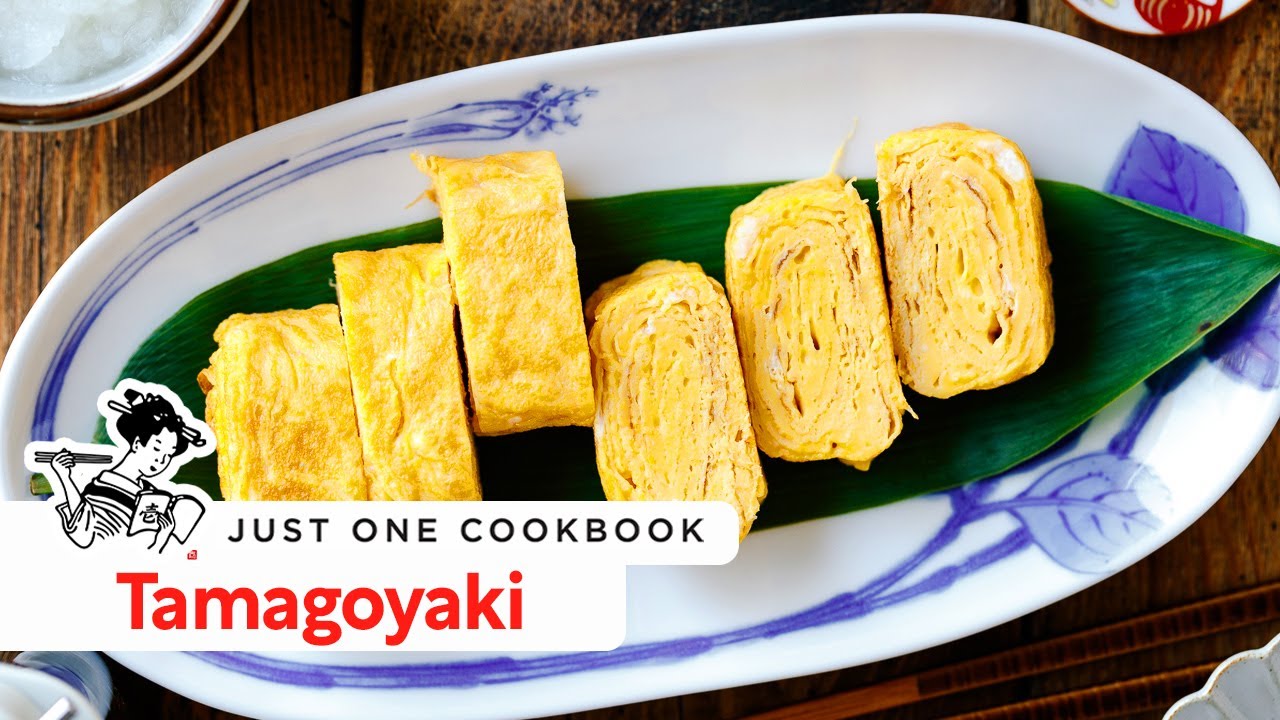The image presents an overhead view of a meticulously arranged oval-shaped, white plate adorned with a blue floral vine design along the edges, set on a dark wooden table. The dish features a long green leaf that stretches across its entire length, serving as a base for six uniform, thick slices of tamagoyaki — a Japanese rolled omelet. The tamagoyaki pieces are densely rolled, revealing their layered, yellow interior reminiscent of an intricately folded pastry. In the bottom left corner of the image, there is a silhouette of a Japanese woman with chopsticks in her hair, reading a book. Next to her, text reads "Just One Cookbook," with "Tamagoyaki" in bold red letters beneath it. The setting hints at other dishes on the table, suggesting a rich traditional meal.